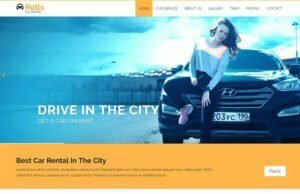The screenshot showcases a webpage from a website named "ROLES," denoted by white capital letters at the top. On the left, there is a black car icon. The image is somewhat blurry but several details are discernable. The website has a navigation menu with six items, the last of which appears to be "Contact." One of the menu items is highlighted in orange.

Below the navigation menu, there is a central image featuring a woman with long hair sitting on the hood of a Hyundai car. She is leaning back against the car, with her right foot against the car's grill and her left foot touching the ground. She is wearing dark pants and a blue blouse, with her left hand resting on her left knee.

Beneath this central image, there is a text caption in white that reads "Driving the city." Further down, there is an orange header box containing the phrase "Best car rental in the city."